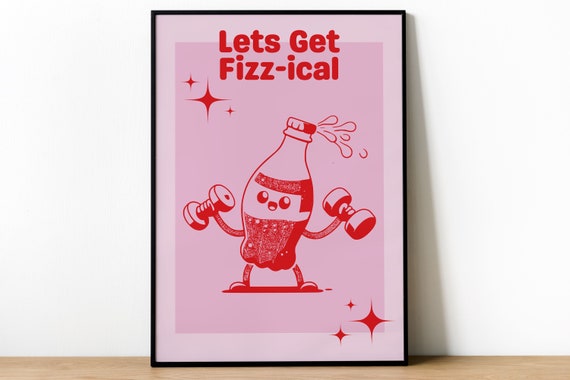This interior photograph showcases a framed, vintage-styled poster staged against a white wall on a natural wood shelf. The illustration within the rectangular poster features an old-fashioned Coke bottle, complete with arms, legs, and eyes, joyfully lifting hand weights to complement the playful caption, "Let's Get FIZZ-ICAL" — a clever play on the word "physical." The vibrant color theme of the artwork predominately consists of lighter and darker shades of pink, with red lettering. Additionally, there are several star-like symbols embellishing the top left corner of the poster. All these elements are neatly enclosed within a thin black frame, adding a touch of elegance to the nostalgic and whimsical design.